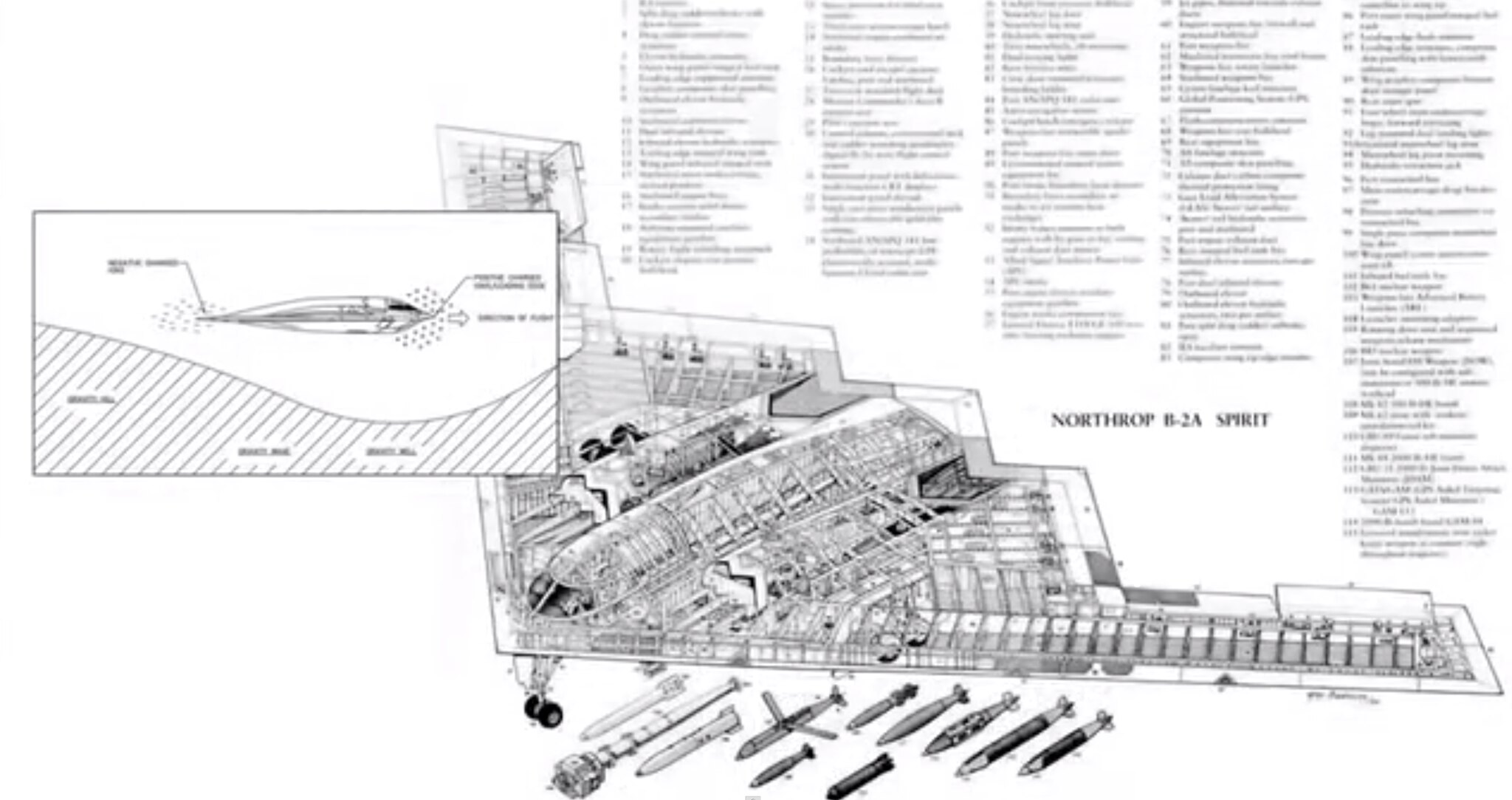The black-and-white image appears to be an illustration from a manual or technical guide, characterized by detailed line drawings and annotated text. The bottom left quadrant of the illustration depicts the inner workings of a complex mechanical structure, potentially a torpedo system or a submarine, based on the context provided. Surrounding this central diagram are several smaller, detailed drawings of individual components, specifically a variety of missiles, extracted for closer examination. The text in the upper right quadrant is arranged in numbered lines, likely serving as references corresponding to various parts of the mechanical structure shown, providing further details or instructions pertaining to each number. Due to the blurred and zoomed-out nature of the text, the specific content remains unreadable.